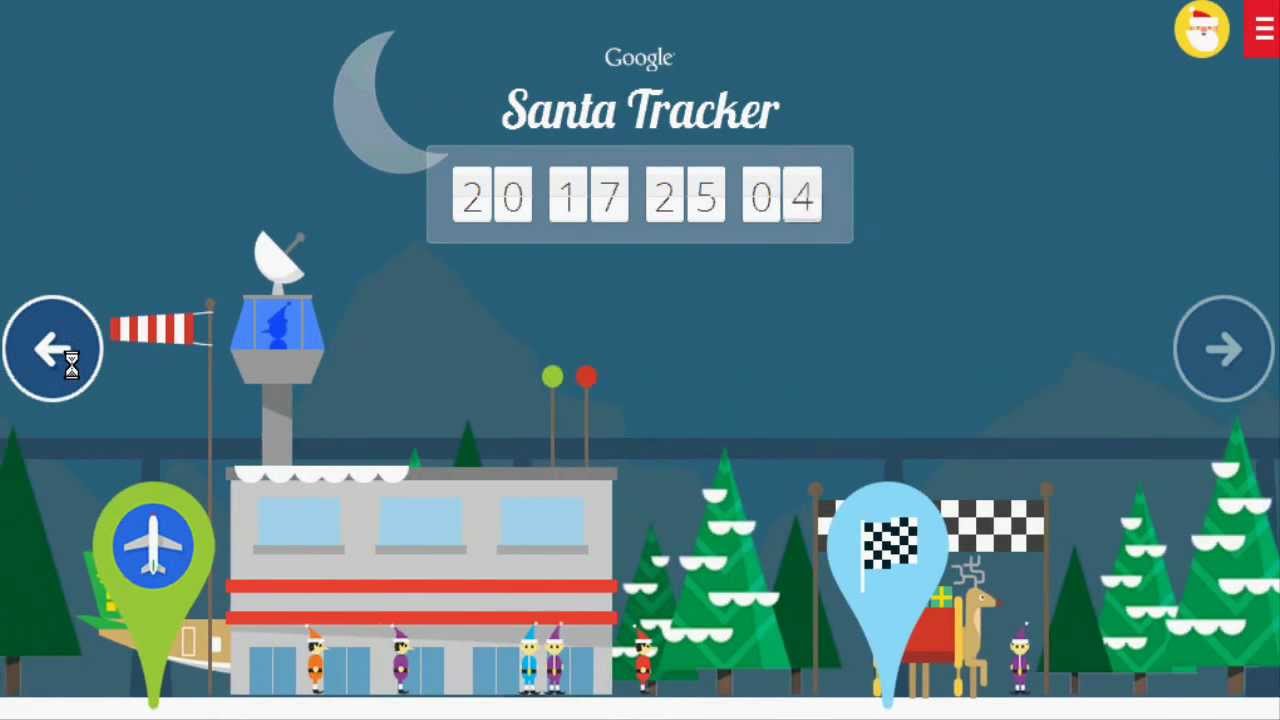The image depicts a Santa Tracker page from Google, featuring a vibrant blue rectangular background. Numerous festive elements are scattered across the screen, including an airplane, a concourse, Christmas trees, and reindeer. In the top right corner, a yellow circle encloses Santa's head, complete with a white beard and a red hat. A red vertical rectangle with three white dashes is also visible.

The webpage prominently displays the title "Google Santa Tracker." A noteworthy visual detail is the depiction of a quarter moon. Below, there are figures reading "2017-2504," followed by a blue horizontal line across part of the screen. Above this line, various items are visible, including a windsock, an unidentified object, a satellite dish, and two lollipop-like figures—one green and one red.

Additional whimsical images fill the space under the blue line, featuring elves, Christmas trees, a winning checkerboard flag, and other festive icons related to the airplane and concourse theme. While the exact purpose of the different elements isn't entirely clear, they collectively contribute to the cheerful Christmas atmosphere of the Google Santa Tracker page.